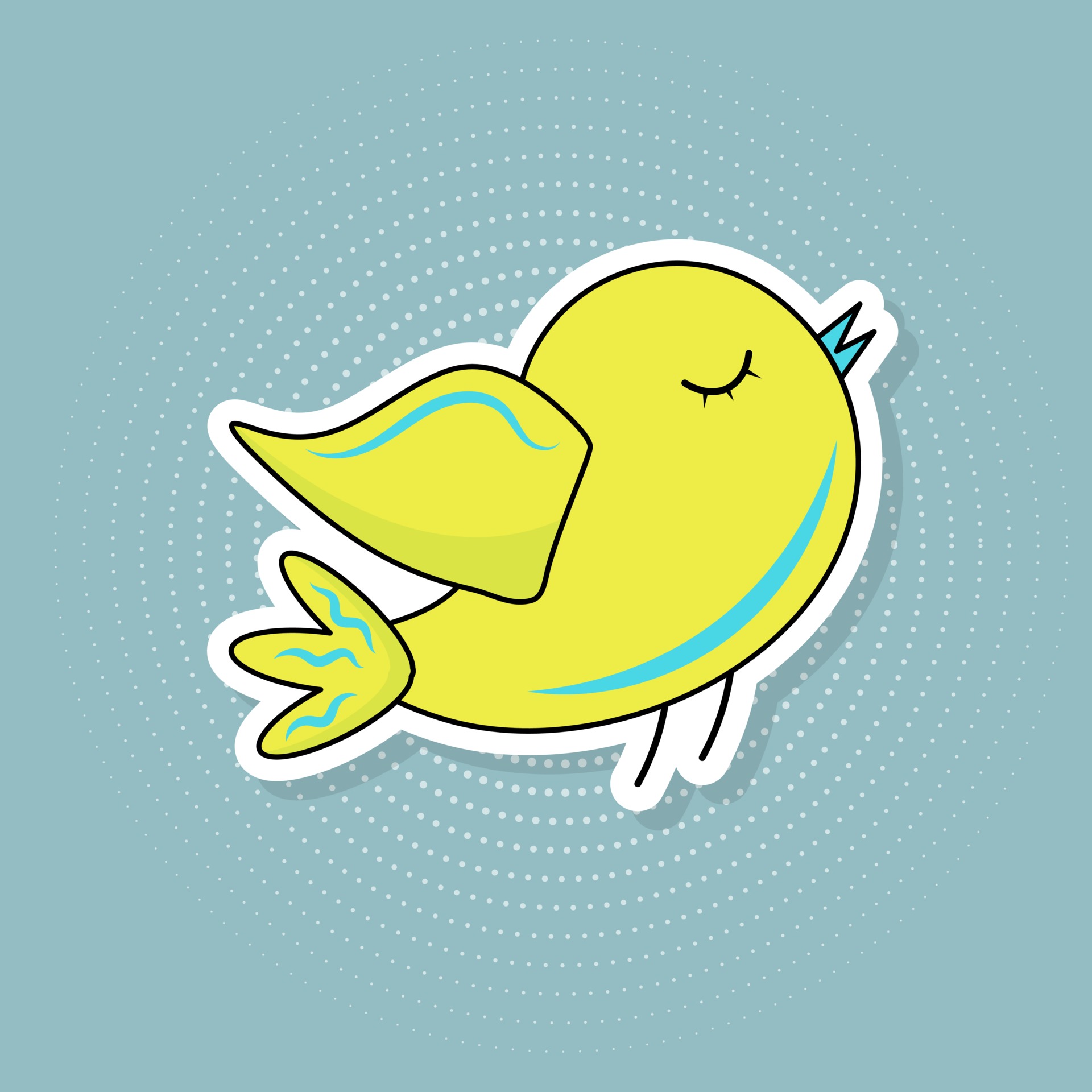This image depicts a cute and stylized cartoon bird, reminiscent of a vector art sticker. The bird, with a plump and cheerful appearance, is yellow with various blue accents, including a blue beak, blue marks under its tummy, and blue highlights on its tail feathers and wing. It is shown in profile, facing to the right with its eyes closed, suggesting a serene or blissful state. The bird is outlined in black with an additional white outline surrounding it. The background is light blue, adorned with several concentric circles of white dots and complemented by squiggly blue lines that accentuate parts of the bird’s wing, chest, and feathery hairs. Together, these elements create a whimsical and lively representation, making the bird appear as if it is joyfully floating in mid-air.